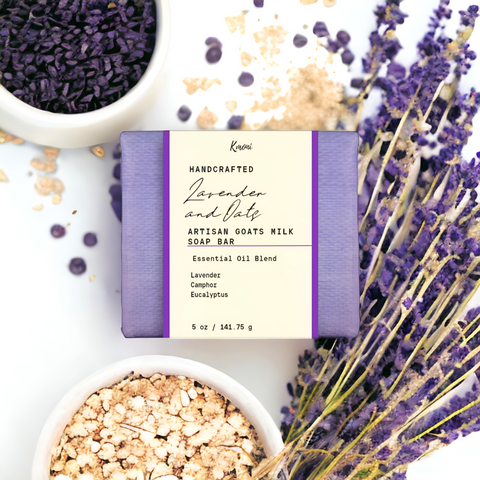This image showcases a detailed and vibrant advertisement for a handcrafted lavender and oats artisan goat's milk soap bar from the brand Kami. The soap, which is wrapped in purple paper with a manila label accented in purple and black lettering, prominently displays the product details: "Handcrafted Lavender and Oats Artisan Goat's Milk Soap Bar, Essential Oil Blend - Lavender, Camphor, Eucalyptus," and notes its weight of 5 ounces (141.75 grams). The setup includes a white tabletop adorned with ingredients featured in the soap, creating an aesthetically pleasing composition. There are bowls containing lavender buds and oats, and scattered around them are sprigs of lavender flowers, oats, and flower petals. The purple of the wrapping paper and lavender elements contrasts sharply with the bright, crisp white background, making the colors and textures of the soap and its ingredients truly stand out.